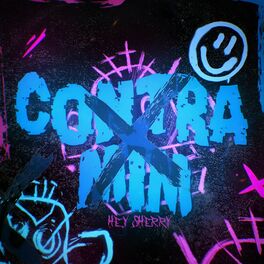Against a stark black background, the focal point of the image features large, vibrant blue letters spelling "Contra MIM," with an X overlaying the text in a slightly darker blue. Below this, in striking pink letters, the phrase "Hey Sherry" is prominently displayed. The upper right corner showcases a silhouette of a smiling face with blue features and a white mouth. The left bottom corner contains lines that ascend up toward the "MIM."

Further enhancing the visual complexity of the scene, the background behind "Contra MIM" boasts pink spikes emerging from a semi-rounded structure. Additional pink streaks are visible at several points: the upper right corner and the right lower corner, as well as a streak shooting up from the right center edge.

The image's vivid colors, reminiscent of a black light effect, give it a glowing quality, as if illuminated by a bright light. Multiple pink faces with exaggerated ears and crosses for hair accompany the text, adding to the overall surrealistic composition. A light blue circle with a simplistic smiley face and line eyes is positioned in the top right, complementing the text and adding a playful touch to the rich and intricate design.